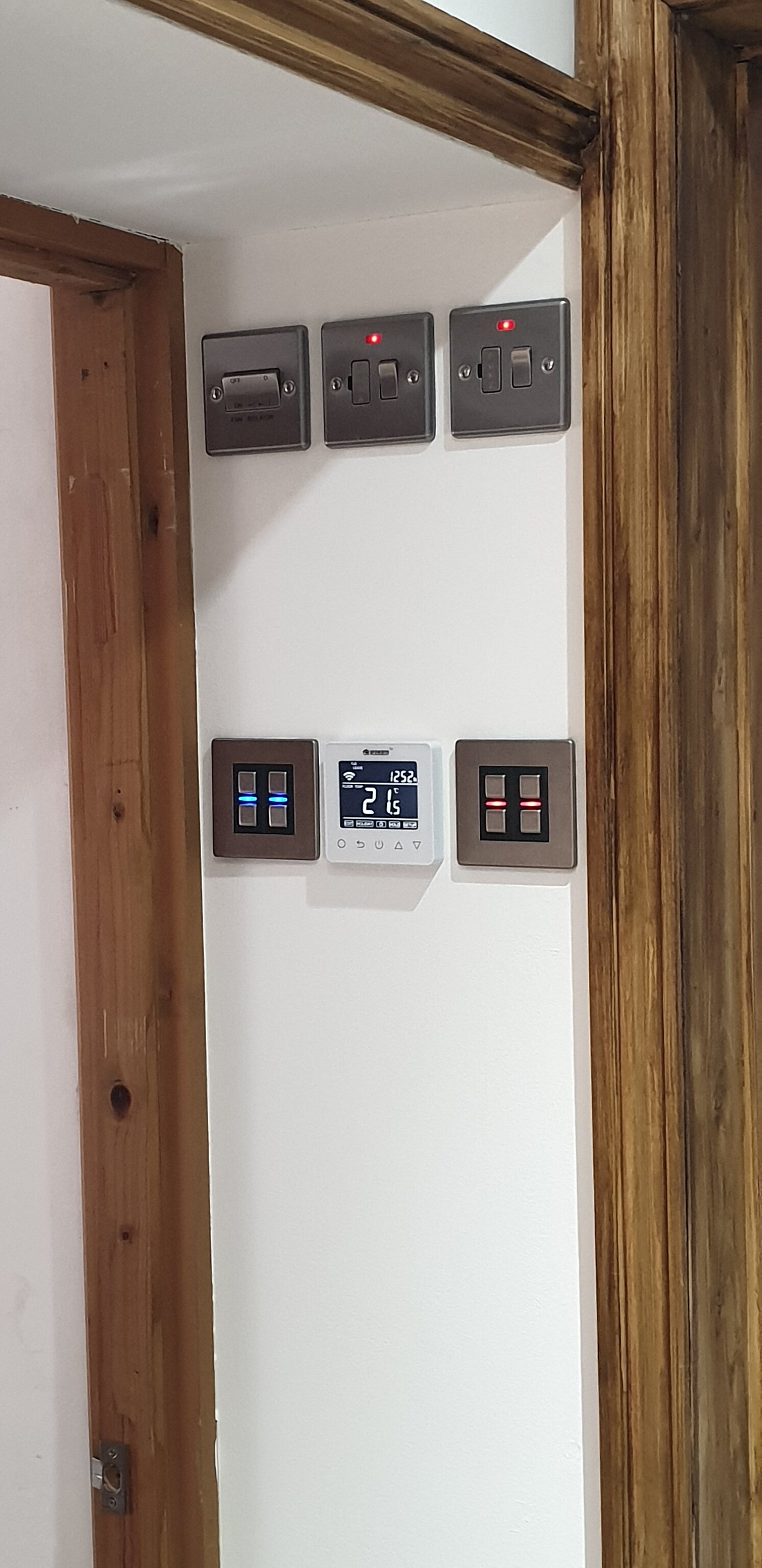The image captures a small, narrow passageway framed by two imposing dark mahogany wooden door frames that stretch high upward. This passage, more reminiscent of a doorway than a complete hallway, lacks an actual door and is bordered by a stark white wall. Attached to this white wall are various control panels and switches. Prominently featured is a sleek, white LED thermostat. Surrounding the thermostat are several metallic, square panels with an array of silver buttons. Notably, two buttons are illuminated in blue, while another two glow red. Above these panels are three square slots, each equipped with silver light switches, two of which have a small red light indicator above them. The image is well-lit, showcasing the bright ceiling that marks the end of the door frame at the top of the picture. The overall atmosphere of the photo is bright and modern.